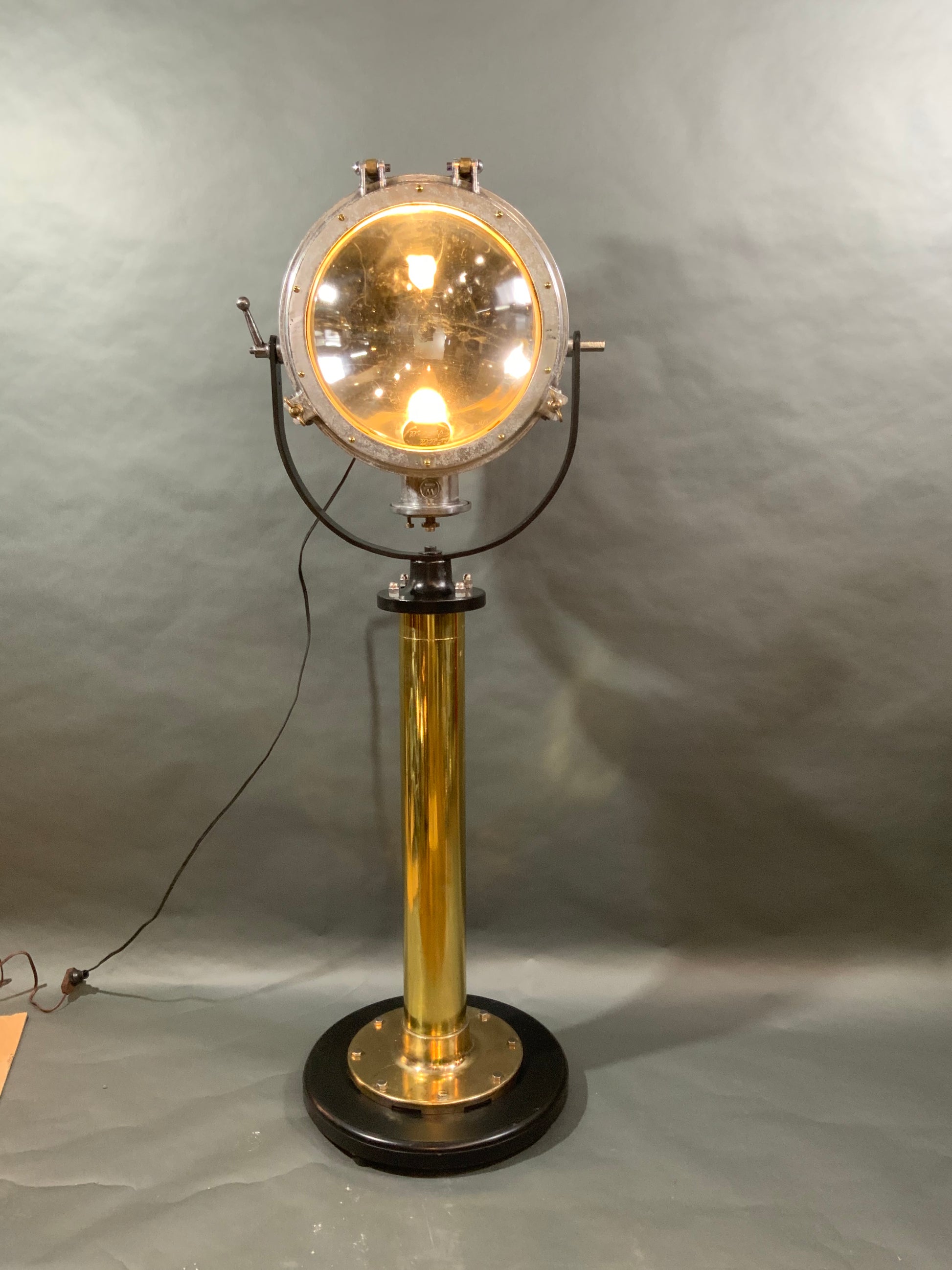The photograph showcases an antique-style lamp that resembles a spotlight, characterized by its distinctive and intricate design. The base of the lamp is round, appearing almost rubber-like, and is topped with a brass faceplate securely fastened with bolts. Rising from the center of the base is a brass pole approximately a foot and a half in height. At the top of this pole, a U-shaped bracket allows for the adjustable positioning of the lamp, enabling it to pivot left, right, up, and down.

The lamp housing is composed of a silver-colored metal with a reflective surface, and encases a domed light bulb at its center. The reflective interior seems designed to enhance the lamp's brightness. A black power cord extends from the back of the housing, draping down towards the bottom left corner of the image. The backdrop of the photograph is a simple gray paper, serving as both the background and the floor, providing a neutral contrast to the lamp's vintage aesthetic.